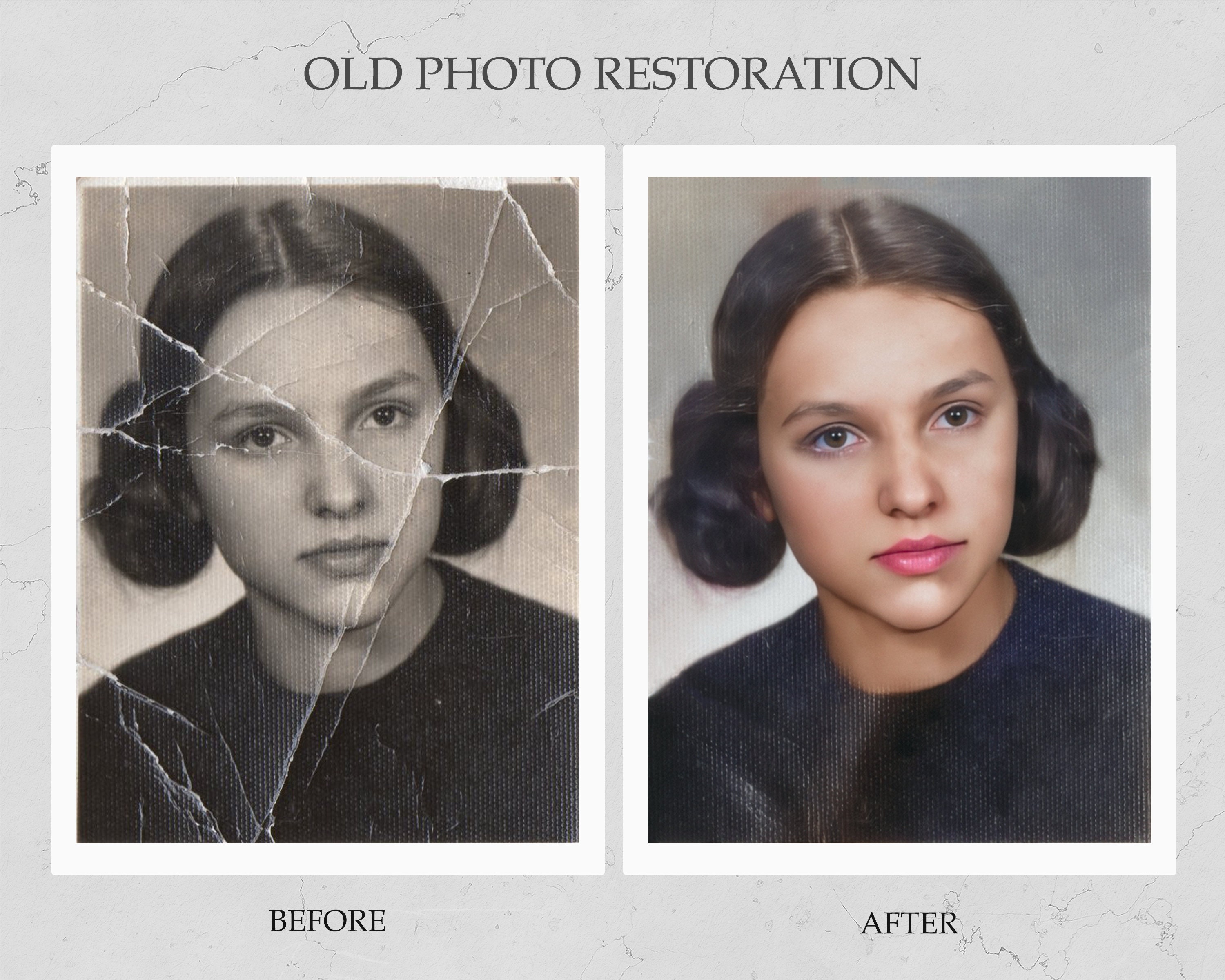This image is an advertisement showcasing historic photo restoration services. At the very top, it reads "Old Photo Restoration." The image consists of two side-by-side photos of the same young woman. The left photo, labeled "Before," is a highly creased black-and-white picture, showing numerous cracks and folds. The young woman, seen from the chest up, has her hair in buns on either side of her face and is wearing a dark shirt. 

The right photo, labeled "After," displays a meticulously restored and colorized version of the same image. The previously visible creases and cracks have been completely eliminated. In this restored photo, the woman has a glowing light to tan skin, brown hair, and hazel or slightly brown eyes. She is adorned with fuchsia pink lipstick, giving a vibrant contrast to her now-colorful and flawless appearance. This side-by-side comparison clearly illustrates the effectiveness of the photo restoration process, transforming a damaged black-and-white photo into a revitalized and colorful image.